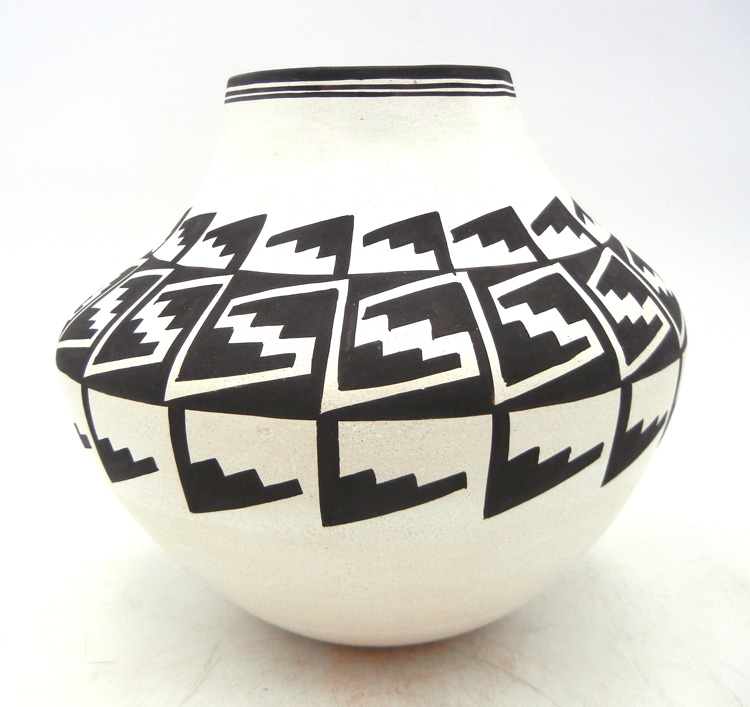This photograph shows a detailed view of a Native American-style ceramic vase from the Southwest, predominantly in black and white. The vase itself is wide and short, with its largest diameter around the center, before narrowing both towards the bottom and the top. Around the top part of the vase, there are three narrow black bands with white spaces in between, decorating the rim. The body of the vase features a repeating pattern that resembles stylized wings, or Z shapes, interspersed around a prominent black stripe which is bordered by white zigzag lines, evoking a staircase-like appearance. This elaborate design runs all the way around the vase, covering the visible 180 degrees. The intricate patterns and alternating black and white imagery create a visually striking piece, reminiscent of stealth bomber shapes and a dynamic, stepped motif.